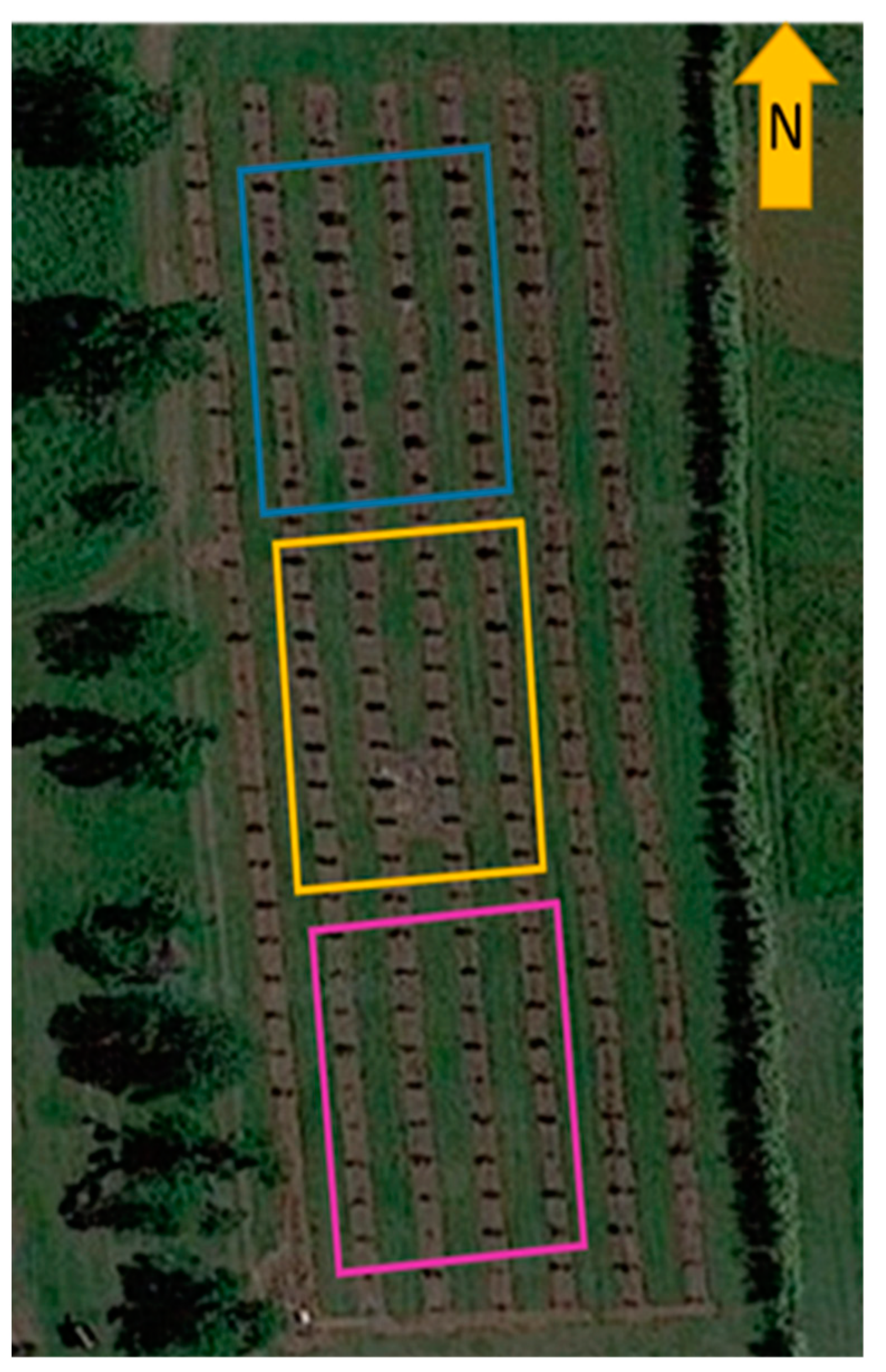This image presents a detailed aerial view reminiscent of a satellite or Google Earth image, displaying a structured and uniform landscape with a notable amount of green areas and trees. The photograph seems to capture a field of crops or a residential block, characterized by seven distinct rows of brown squares running vertically, which could be identical houses or uniform plots of land. Each column within these rows contains roughly 20 small squares. Surrounding the field are sections of green, likely grass, interspersed with darker shading indicative of trees along the sides, with a hedgerow on the right.

Adding to the organized layout are three digitally imposed rectangular boxes, each in a different color: a blue rectangle at the top, a yellow rectangle in the center, and a magenta or fuchsia rectangle near the bottom. These boxes highlight specific sections of the rows, with the purpose of these markings remaining unclear. Additionally, a gold arrow pointing upwards, located in the top-right corner and labeled with the letter "N," indicates that the image is oriented with the top pointing north. The overall composition suggests an image taken from a significant altitude, capturing the intricate details of the land below.